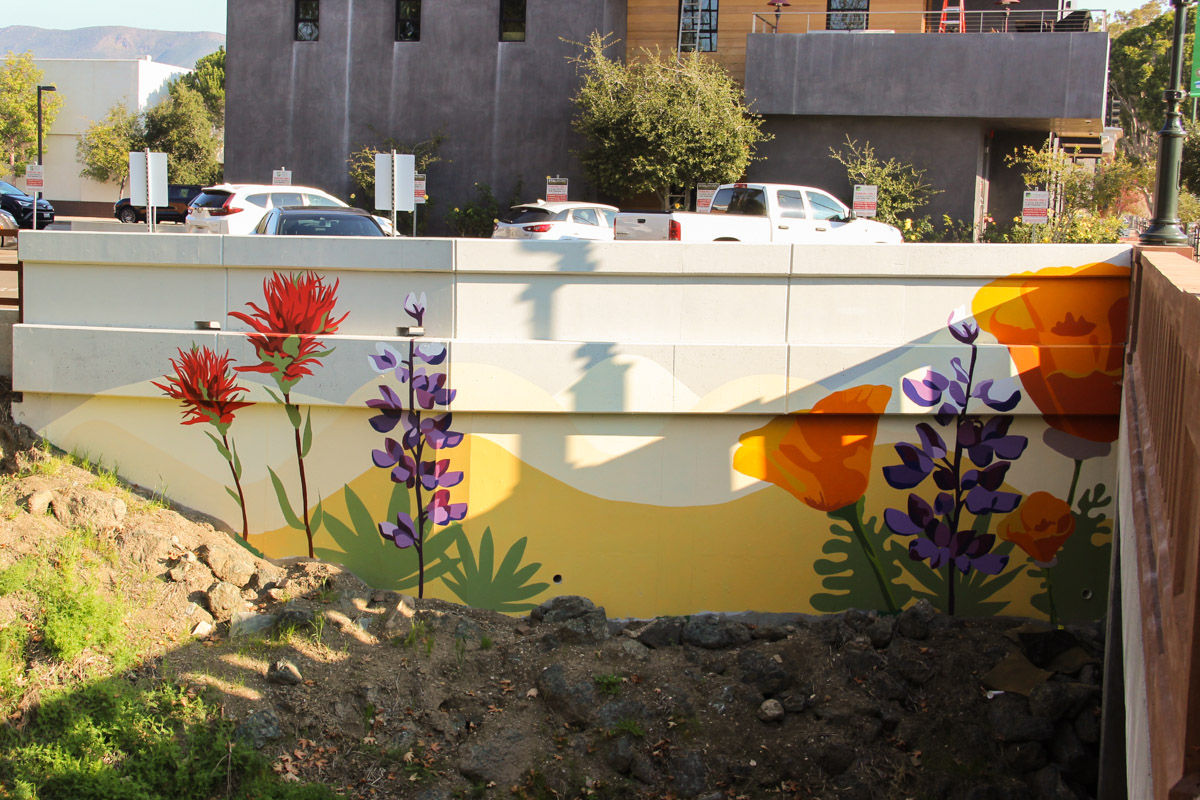The image depicts a vibrant outdoor scene dominated by a white painted concrete wall adorned with murals of red poppies, purple lavenders, and minimalistic shapes, including a yellow silhouette of mountains in the background. Below the wall is a patch of brownish dirt with scattered rocks and a grassy area to the left. The sunlight bathes the entire scene, creating reflections and highlights on the wall and surrounding objects. To the right, a normal brown fence is visible, and beyond it, a parking area is lined with cars, a gray concrete building with wood paneling, and various street signs and light poles. In the distance, a mountain range stretches under a bright blue sky. Additionally, there are trees along the parking area, and a construction site featuring a two-story concrete building. An old bridge adds to the rich, textured landscape captured on this sunny day.